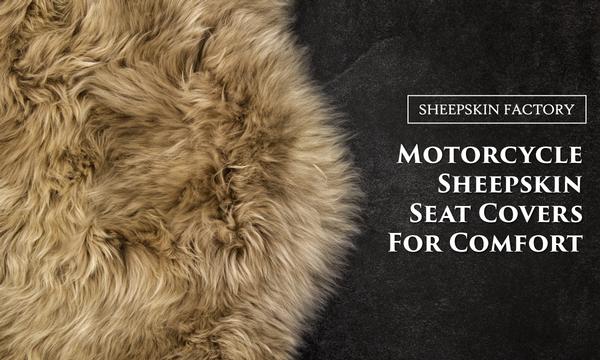This advertisement image is split into two halves. On the left, there is a vibrant, landscape-format depiction of soft, brown sheepskin with long and fluffy fur, resembling a shag rug. This sheepskin cover evokes a sense of comfort with its luxurious, furry texture, implying it could be used for motorcycle seat covers. The right side of the image features a black background with a paper-like texture. Here, the white text "Sheepskin Factory" is enclosed in a white outlined square at the top, emphasizing the brand. Below it, in big white letters, it reads, “Motorcycle Sheepskin Seat Covers for Comfort,” highlighting the product's function and quality. The overall color scheme of the ad is black, white, and brown, and the lighting seems to come from above, making the image very vibrant and bright.